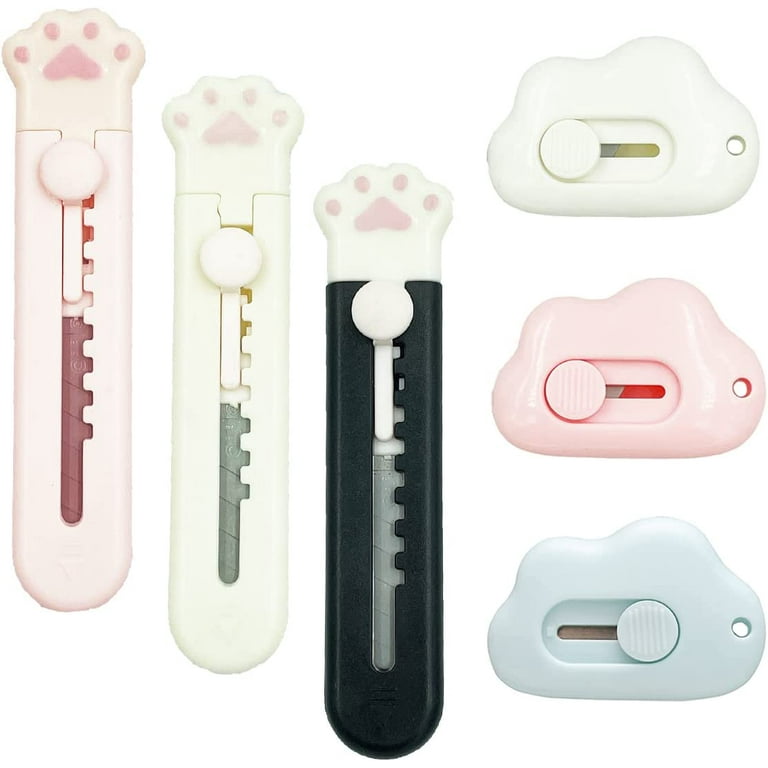The image features a set of three distinct handle tools against a solid white background, characterized by their unique design resembling an animal paw print at the rounded tip. Each handle is equipped with a colored insert seen through a central groove, suggesting adjustable functionality. The left handle is light pink with a dark red backing, the middle one is white with a green backing, and the one on the right is black with a gray backing. These intricate tools also showcase a close-up section to the right, displayed vertically, highlighting the detailed design of the rounded, paw print-like tip in light pink, white, and blue. This close-up shows a circular knob, which appears to allow adjustment or activation, reinforcing the functional aspect of the handles, much like retractable instruments.